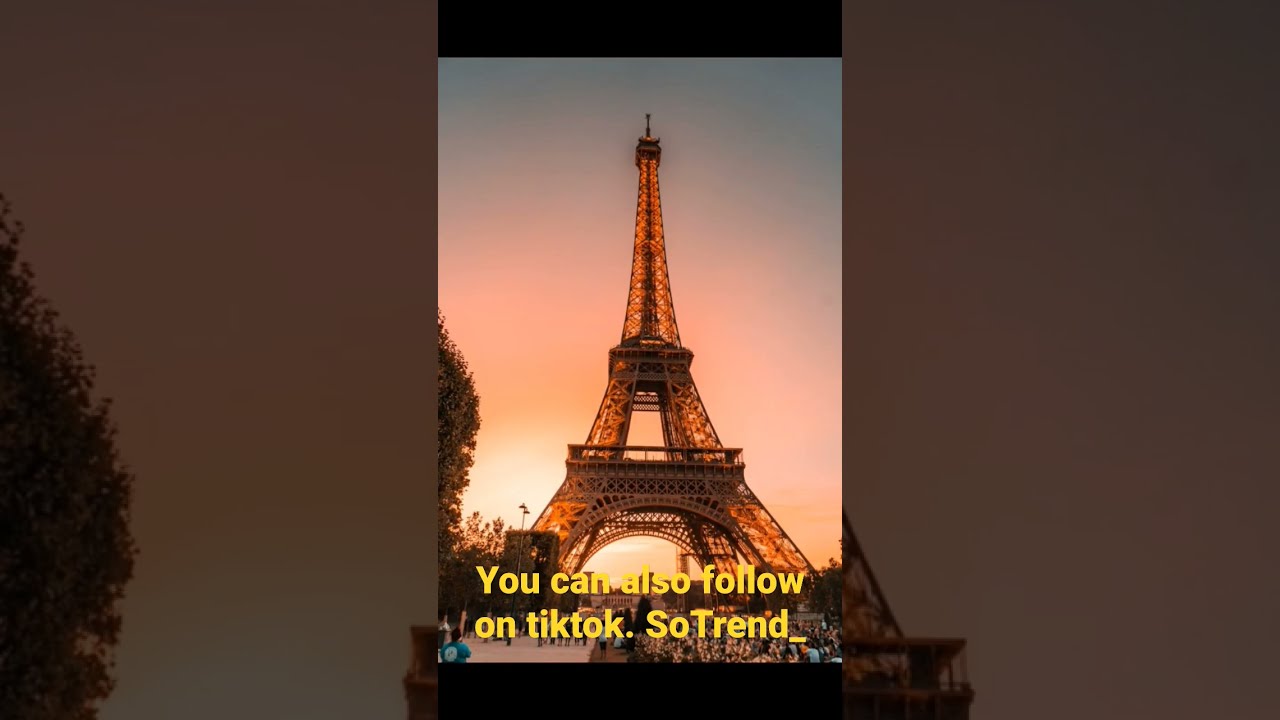The image captures the Eiffel Tower at sunset or sunrise, taken vertically from the ground upward with a smartphone. The iconic tower glows with an orange and yellow hue, thanks to subtle internal lighting, creating a striking silhouette against a backdrop of a cloudless sky that transitions from orange and pink at the base to blue at the top. At the bottom of the photo, there is a paved area where people are milling about, along with the partial view of a tree with leaves extending from the left and a light pole. The scene includes a small structure also on the left side. Notably, the photo features a larger, faded duplicate of itself laid in the background. A black stripe borders the top and bottom of the picture, with the bottom stripe highlighting yellow text that reads, "you can also follow on TikTok @sotrend."